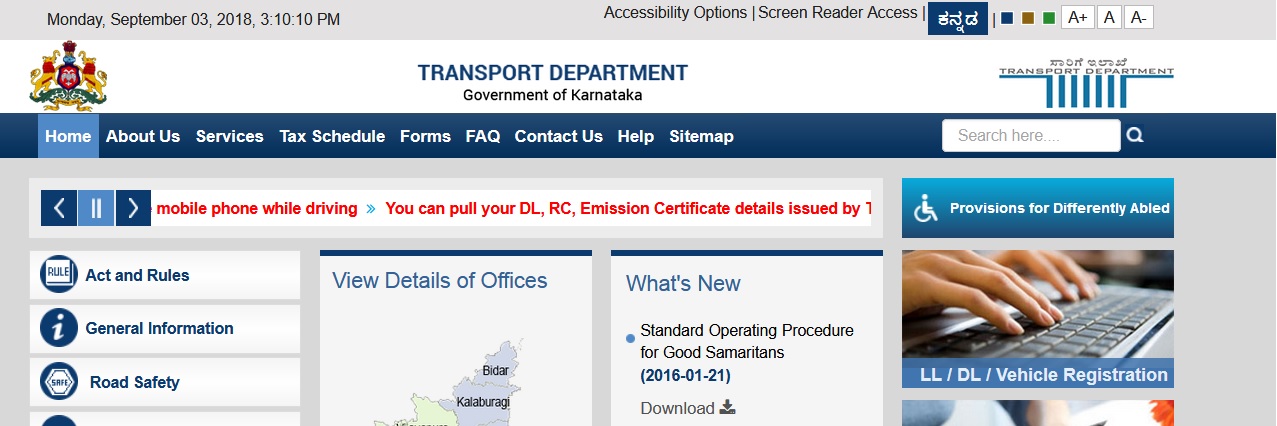The image depicts a section of the official website of the Transport Department, Government of Karnataka, captured on Monday, September 3, 2018, at 3:10 p.m. At the top, there are accessibility options, including Screen Reader Access, ensuring the site is usable by all individuals. The logo of the Transport Department is prominently displayed, featuring two animals, likely elephants, flanking a shield, reminiscent of a medieval-style family crest.

Navigational links on the site include Home, About Us, Services, Tax Schedule, Forms, FAQ, Contact Us, Help, and Sitemap, providing structured access to various sections of the website. A notable banner in blue with red lettering warns about the dangers of using a mobile phone while driving. The banner also mentions that users can pull up details such as their Driving License (DL), Registration Certificate (RC), and Emission Certificate, although the text is partially cut off.

The website features sections dedicated to Acts and Rules, General Information, and Road Safety. In the middle portion, there is an interactive map highlighting details of various offices, with specific mentions of locations like Bidar and Kalaburagi, indicating the site is likely centered around India.

In the "What's New" section, there is an update titled "Standard Operating Procedure for Good Samaritans" dated January 21, 2016, with a downloadable link provided. To the right, there is a segment for "Provisions for the Differently Abled" showcasing an illustration of hands at a keyboard. This section also mentions LLDL Vehicle Registration, reinforcing that this is a motor vehicle administration website. The site is in English, suggesting it is accessible to a broad audience.